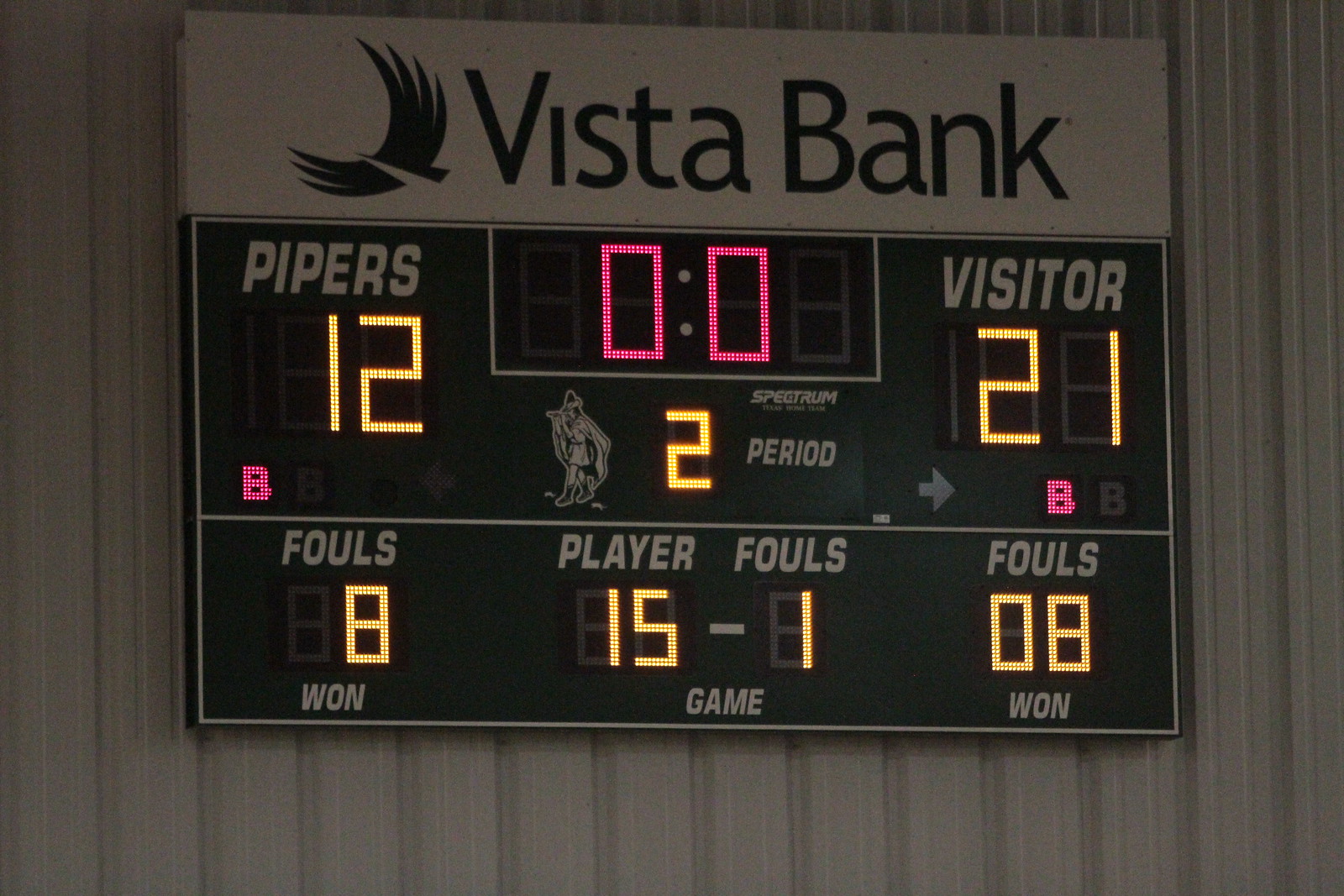This is a detailed photograph of an electronic scoreboard mounted on a white wall featuring intersecting line patterns. At the top of the scoreboard, it prominently displays "Worcester Bank," accompanied by a bird logo situated to the left of the bank name. The top section of the scoreboard has a white background, while the area below transitions to a black background, divided into two main rows.

On the first row of the black background, the left side reads "Pipers 12," indicating the home team's score, with an illuminated "0-0" clock in the middle. Below the clock, it reads "2," signifying the second period of the game. The right side of this row shows "Visitors 21," denoting the opposing team's score.

The second row, dedicated to fouls, begins with "Fouls" on the far-left side under "Pipers," with numbers "8-1" illuminated below. The middle section states "Players Fouls" with "15-1" displayed beneath it. On the far-right side, under "Visitors," it lists fouls as "0-8-1." The scoreboard also features a small mascot logo of the Pied Piper centrally located beneath the period indicator.